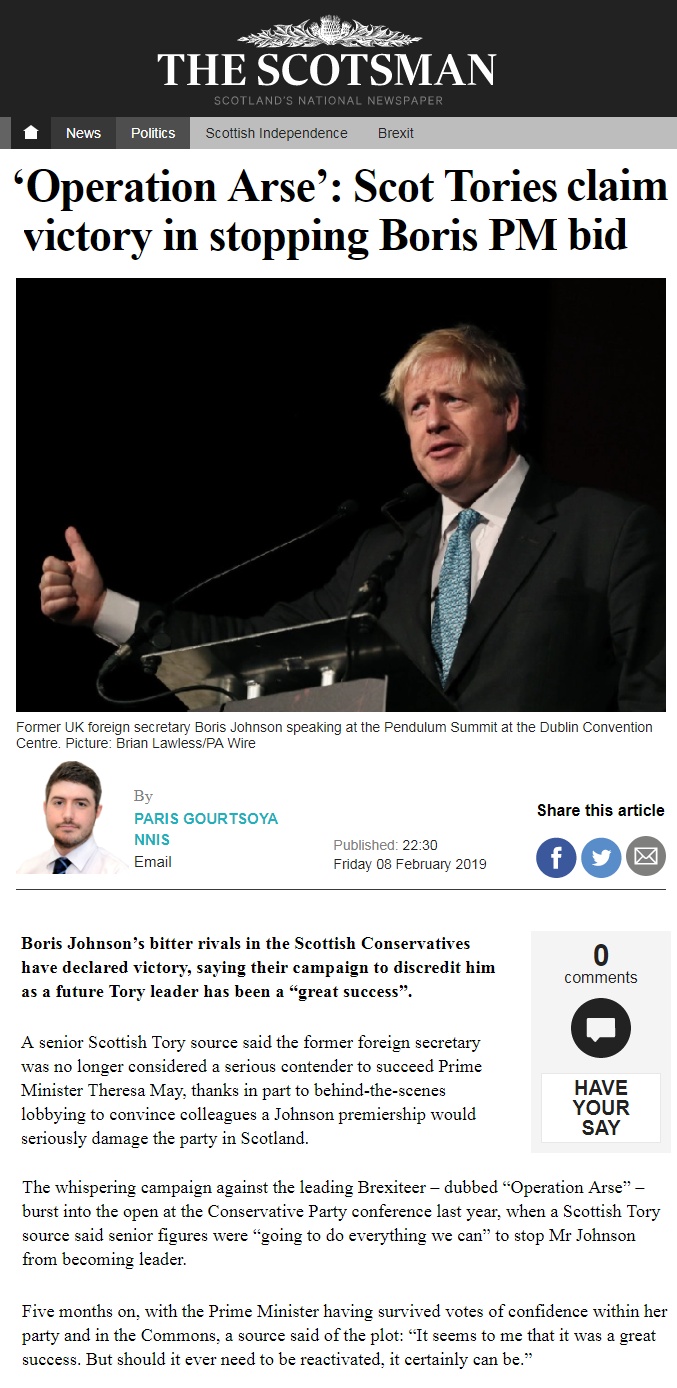This image is a vertical screenshot of an article from The Scotsman, Scotland's National Newspaper. The top black horizontal bar features the bold white text "THE SCOTSMAN" in all caps, with a white thistle logo and some leaves above the title. The menu bar below indicates options such as News, Politics, Scottish Independence, and Brexit. Underneath, the background is white.

The headline, presented in bold black letters, reads: "Operation Arse: Scott Tories claim victory in stopping Boris PM bid." Below the headline is a horizontal landscape photograph of Boris Johnson. He is standing in front of a lectern, dressed in a suit with a blue tie, and giving a thumbs-up gesture. The photo caption notes: "Former UK Foreign Secretary Boris Johnson speaking at the Pendulum Summit at the Dublin Convention Centre, Picture Brian Lawless/PA Wire."

The article is authored by Paris Gortz Soya and is timestamped at 22:30 on Friday, 06 February 2019. The piece details how Boris Johnson's rivals within the Scottish Conservatives have declared their campaign to discredit him as a future Tory leader a significant success.